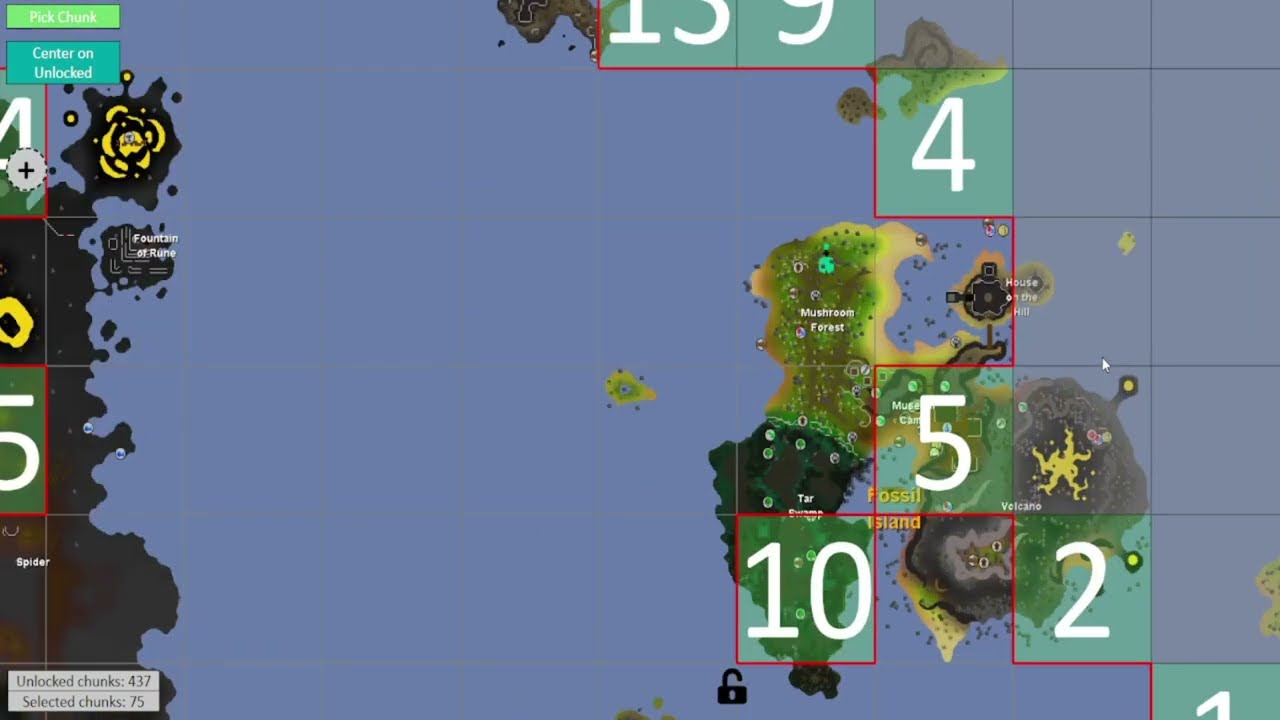The image is a detailed map from the video game RuneScape, showing a large expanse of ocean with various landmasses primarily on the right. A grid pattern overlays the map, with numbered squares such as 5, 2, 10, and 4, and several empty boxes, particularly in rows. Notable locations labeled on the map include "Fossil Island" in the bottom-right area and "Wilderness" along the left side. Additionally, the map features names like "Mushroom Forest" and shows a volcano. At the top left of the image, there are selectable boxes labeled "Pick Chunk" and "Center on Unlocked," while the bottom left shows "Unlocked Chunks 437" and "Selected Chunk 75." The grid and numbers suggest that this is a strategic or exploration mechanic within the game, emphasizing the detailed and navigable areas such as Fossil Island and the surrounding regions.